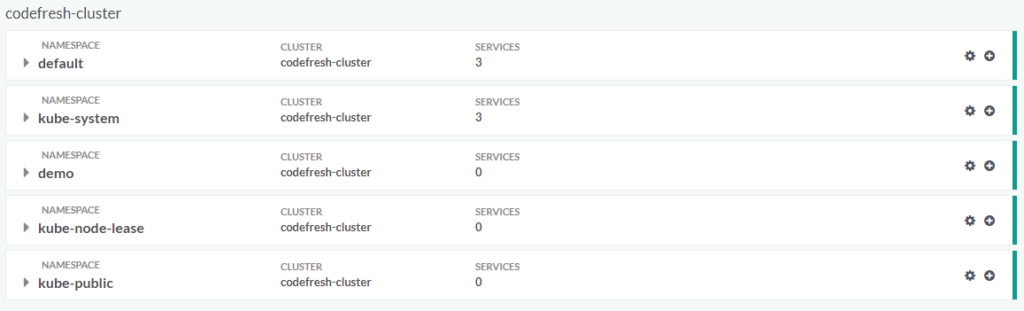The image features a horizontally oriented layout dominated by white rectangles set against a backdrop of a very light greenish-blue hue. Each white rectangle contains detailed information presented in a dark charcoal gray or black color for clear visibility.

At the top, bordered by a slim margin, the title "CodeFresh-Cluster" is prominently displayed. Directly below it, spanning the width of the rectangle, is the first information box that reads: "Namespace: Default, Cluster: CodeFresh-Cluster, Services: 3," and concludes with two icons and a green line.

Sequentially listed beneath this initial box are additional namespaces with similar structures. The second one states "Namespace: kube-system," followed by "Namespace: demo," "Namespace: kube-node-lease," and "Namespace: kube-public." Each namespace box to the right aligns under the cluster designation "CodeFresh-Cluster" and includes a services section. The first two namespaces list three services each, while the remaining namespaces indicate zero services. Each box concludes uniformly with the same two icons and a green line, mirroring the design of the first.